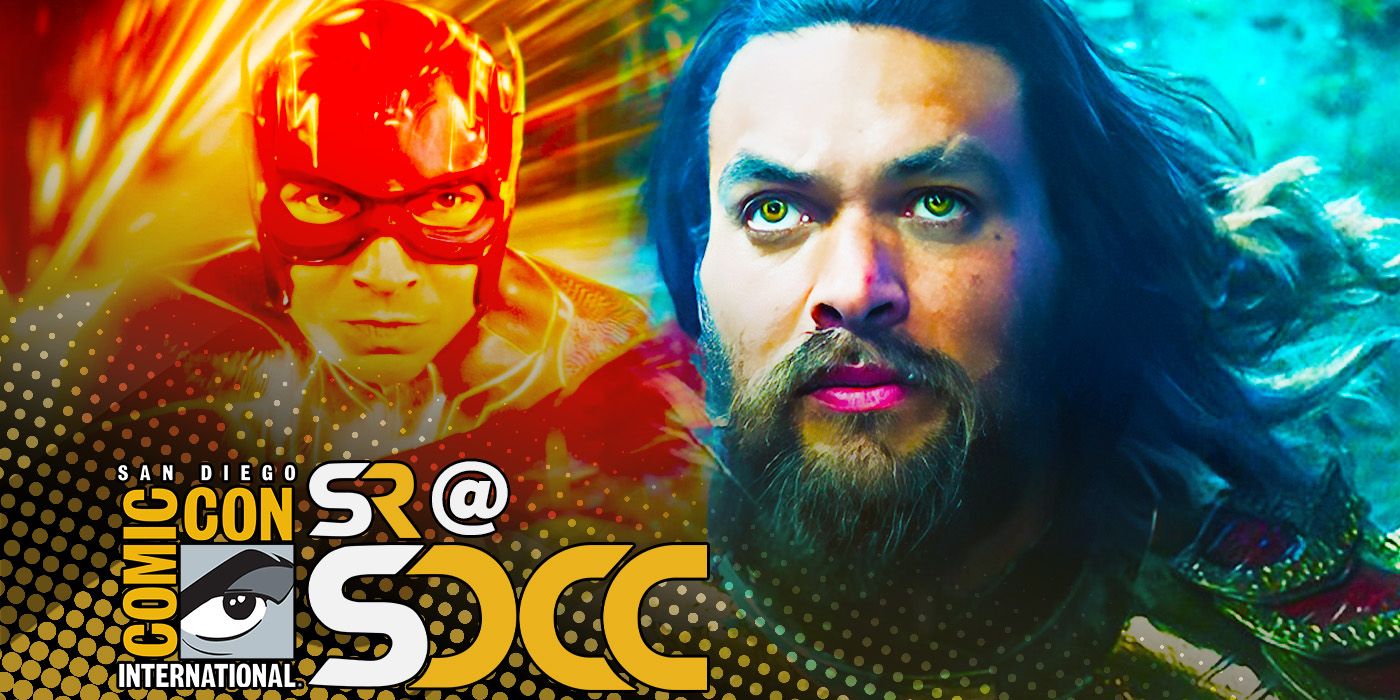This visually striking promotional poster for San Diego Comic-Con International features a dynamic split-image design. On the left side, we see The Flash, portrayed by Ezra Miller, in his iconic red suit, surrounded by a background of vibrant red and yellow lights that evoke a sense of speed and energy. In contrast, the right side showcases a zoomed-in, contemplative image of Aquaman, played by Jason Momoa, set against a blue underwater background that highlights his rugged, bearded look and piercing gaze. The Comic-Con logo is prominently displayed in the bottom left corner, featuring a gray square with an eye, along with the text "SR at SDCC" in a mix of white and yellow fonts. The poster is overlaid with a diagonal dotted grid, adding a modern, tech-inspired aesthetic to the composition.